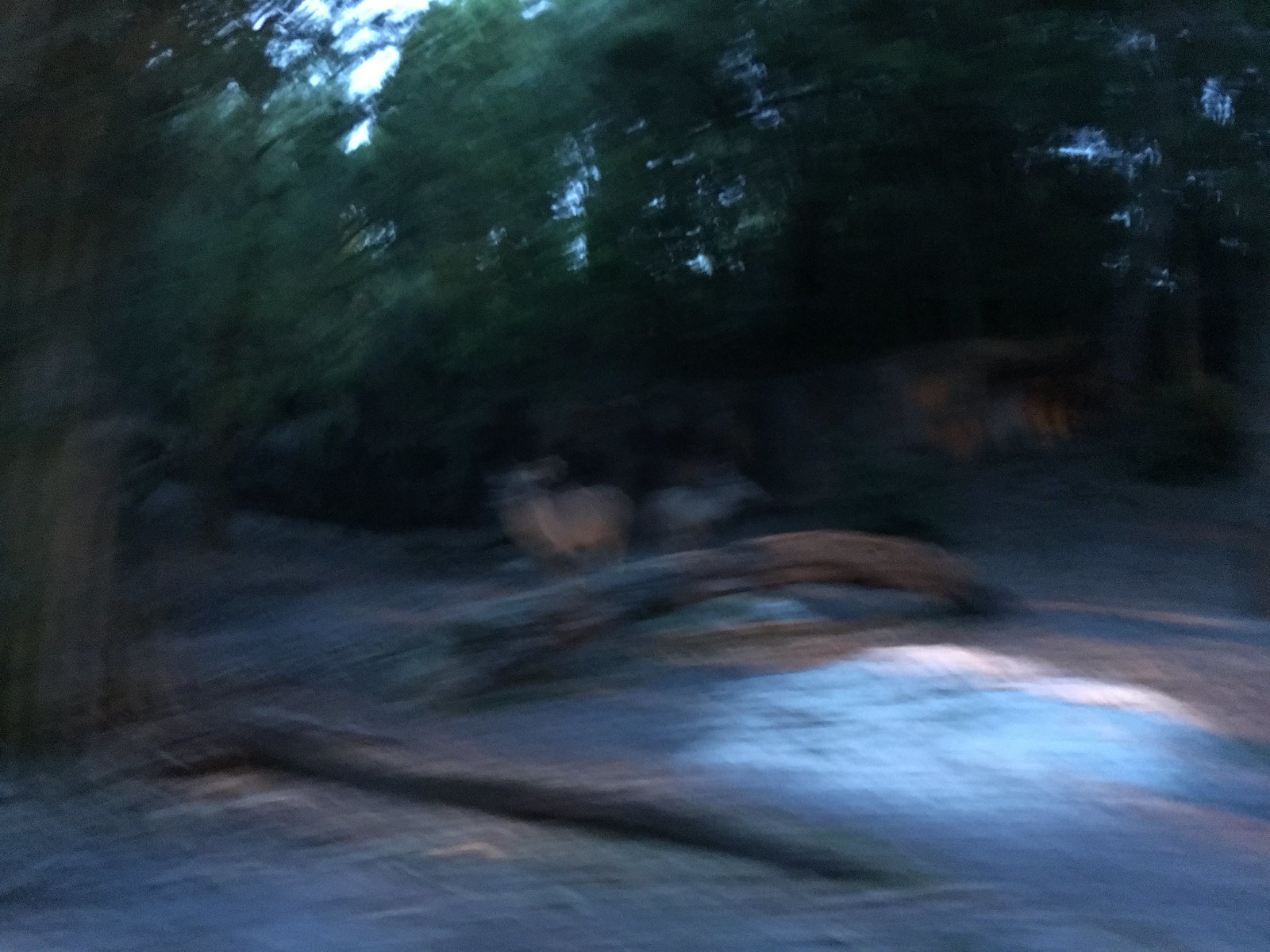This photograph captures a forested setting, possibly a roadside park or an outdoor backyard, bathed in the soft light of early evening. Despite the image being notably blurry, several key elements can be discerned. Centrally located, three to four deer are visible, with two of them partially obscured by a fallen tree that exhibits a gentle curve. This tree, lying across what appears to be a dirt path or road, serves as a natural barrier in the scene. The presence of faint headlights or a flashlight beam illuminates the foreground, suggesting human activity nearby. The sky above is a bright blue with scattered clouds, contrasting with the dimly lit environment below. Surrounding the deer are additional fallen trees, reinforcing the rugged, natural aspect of the area. This composition evokes a tranquil, if slightly mysterious, slice of wilderness life.